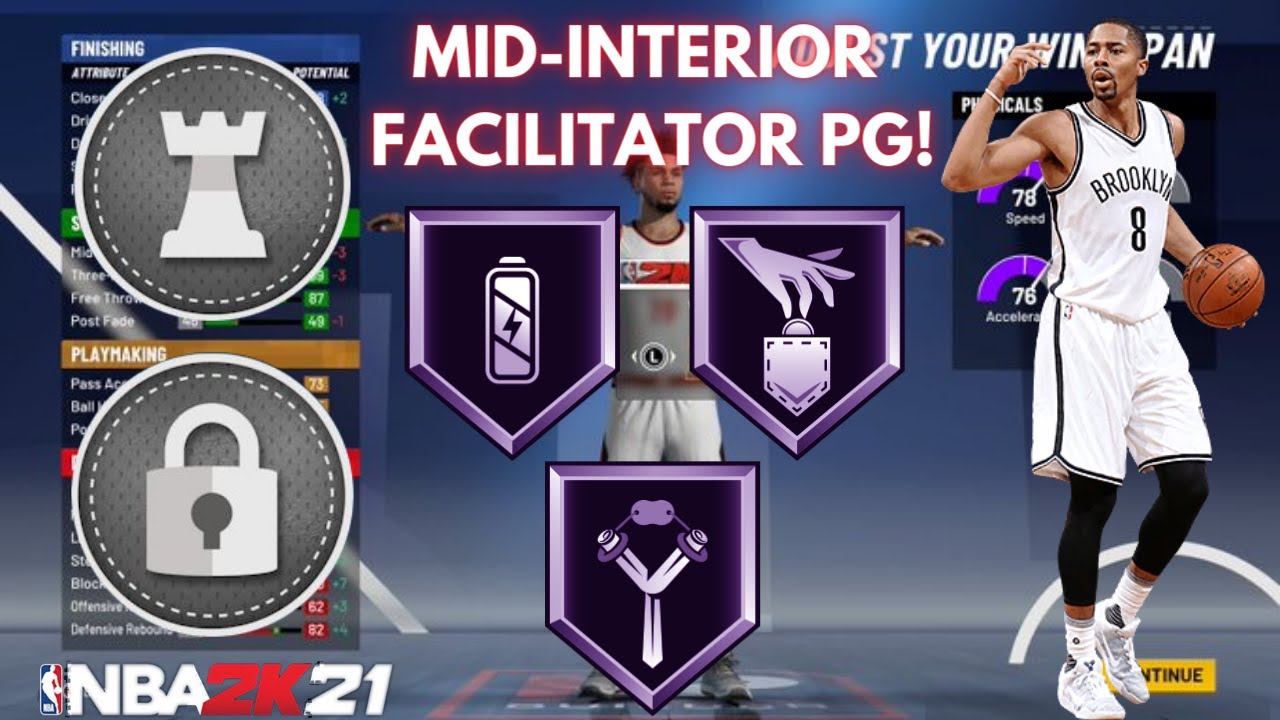This promotional image for the video game NBA 2K21 highlights a specialized character build known as the "Mid-Interior Facilitator" for the Point Guard (PG) position. Centered on the image is a dynamic illustration of a basketball player wearing jersey number 8 from the Brooklyn Nets. The player is captured mid-dribble, exuding an intense focus as he prepares to make his next move.

Dominating the background, the main text in bold white font reads "Mid-Interior Facilitator PG," indicating the specific role and attributes of this player build. The image features three prominent badges, each within a purple shield-like frame, signifying their high-level importance. Badge 1 is symbolized by a battery icon, possibly representing endurance or energy. Badge 2 features a hand with a lock, likely indicating superior stealing abilities. Badge 3 depicts a weightlifting icon, suggesting enhanced strength or physical conditioning.

On the left side of the image, two circular icons appear: one with a castle rook (chess piece) and another with a padlock, which could denote locked or protected abilities. The lower left corner of the image displays the official NBA 2K21 logo, ensuring clarity on the game being referenced.

In the background, character stats can be faintly seen, highlighting attributes such as speed and acceleration, further emphasizing the customization and depth available in creating a player build within NBA 2K21. Overall, this image aims to present a nuanced and powerful player archetype, offering gamers a strategic edge on the virtual basketball court.